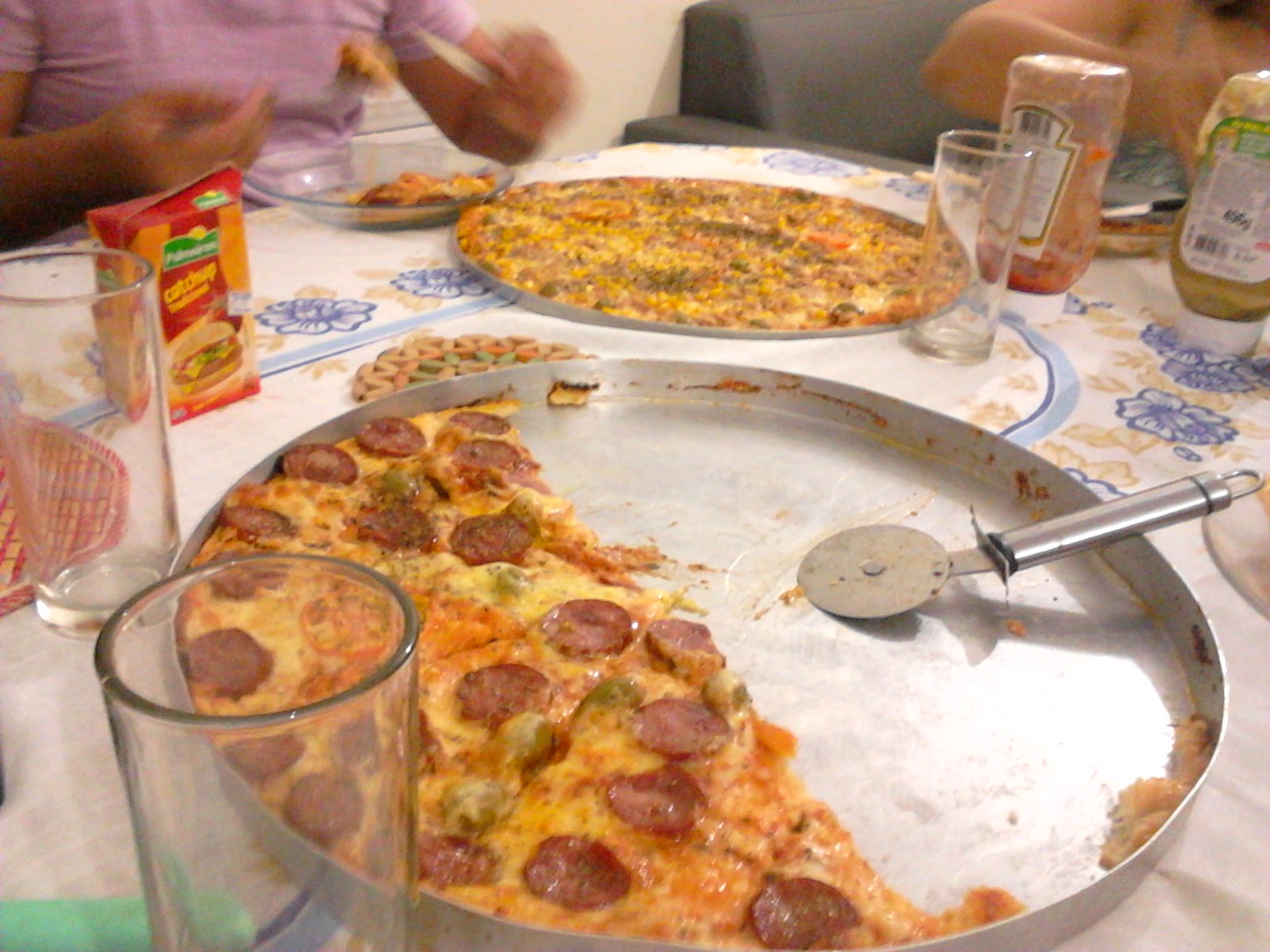The photograph captures a lively gathering around a white, felt-backed plastic tablecloth adorned with blue flowers. At the center of the table, two large tin pans hold pizzas. The pizza closest to the camera is a half-eaten pepperoni pizza, with four slices remaining on the right side and a pizza wheel resting in the empty silver space on the left. The other pizza appears untouched, its toppings perhaps including ham, cheese, and something brown. Around the table, there are several clear, empty glasses along with bottles of ketchup and mustard situated at the top left of the table.

In the background, a person wearing a pink shirt is visible, eating with a knife and fork from a glass plate. To their left, a gray couch and another person’s bent elbow, also clad in pink, can be seen. Before this second person lies a thin layer of taco dip, possibly containing meat, corn, and tomatoes. The cozy, detailed setting suggests a warm, casual gathering where everyone is enjoying a pizza meal together.